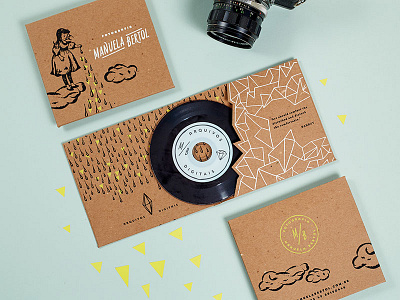This is an overhead color photograph featuring a carefully arranged vinyl record and its packaging, set against a light robin blue background adorned with downward-pointing yellow triangles. At the top of the image, partially cut off, is the black lens cap with a silver band of a camera. The composition focuses on an album cover for Manuela Bertol. The cover, in a brown hue, showcases an old-fashioned pen-and-ink styled sketch of a girl in a dress standing on a cloud, letting black and yellow drops of liquid fall from her hand. Encircling this scene are more yellow triangles. The open album cover in the center reveals a pocket with a white fractal sketch, containing the black vinyl record with a white label and an additional diamond icon sketched on it. The bottom part of the image depicts the back of the record packaging, featuring a simple illustration of three clouds similar to the ones on the front. The text on the record label is too small to read, emphasizing the visual artistry of the album design.